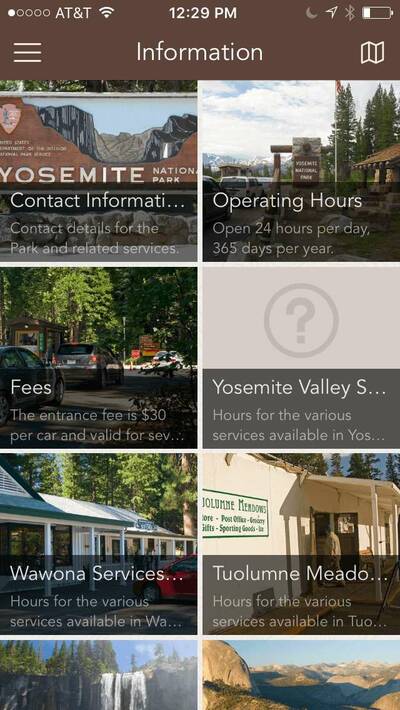Screenshot of an older iOS interface on an iPhone displaying a website about Yosemite National Park. The top-left corner of the screen shows five round signal indicators, with only one circle filled, indicating poor reception. Next to it, "AT&T" is displayed, followed by three Wi-Fi bars, and the time "12:09 PM" centered. Further to the right, several icons are shown, including a grayed-out moon icon, a location icon, a grayed-out Bluetooth icon, and a battery icon indicating approximately 20-30% charge remaining.

On the left side below the top bar, there are three horizontal lines stacked (likely a menu icon), while the center displays a title, "Information," with a capital "I." On the far right, a map icon is present. The top border of the page is brown, beneath which the screen is divided into a grid of two columns and four rows of image tiles.

**First Row:**
1. **Contact Information**: Displays contact details for the park over a background featuring a mountain range with the text "Yosemite National Park."
2. **Operating Hours**: States "Up to 24 hours per day, 365 days per year" and features an image of the park's entrance with tall pine trees and white clouds in the sky.

**Second Row:**
1. **Fees**: Mentions the entrance fee of "$30 per car" and shows cars with red taillights on along a tree-lined road. The text gets cut off but continues on the next row.
2. **Yosemite Valley Services**: Describes hours for various services available in Yosemite Valley. The background is plain gray with a light gray circle and a question mark.

**Third Row:**
1. **Wawona Services**: Provides hours for various services in Wawona, displaying an image of a building with white pillars, a wide roof, green trees, and a red car parked outside.
2. **Tuolumne Meadows**: Describes services available in Tuolumne Meadows, showing a white building with an open door. A man is seen walking into the building, with trees in the background and a green-bordered sign listing offerings such as post office, grocery, and sporting goods.

**Fourth Row:**
1. An image partially visible, showcasing a waterfall with blue skies, tall green pine trees, and cascading white water.
2. Another partly visible image, showing an aerial view of a mountain range with brown and gray tones, under sunlight.